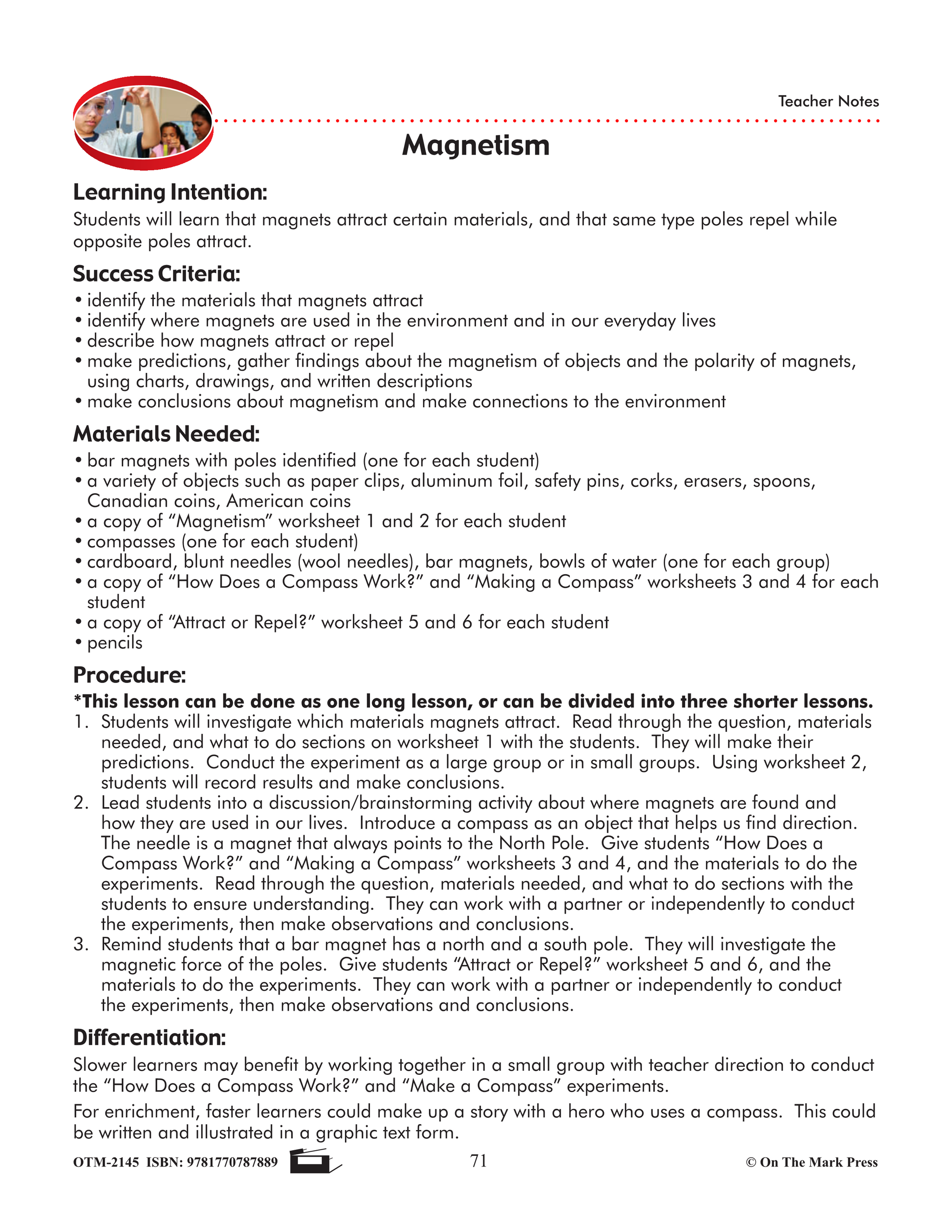This image is a full page from a textbook or teacher's edition detailing a science experiment on magnetism. The page has a white background. In the top left corner, there is an oval picture bordered in red, showing three children in a classroom setting engaged in a scientific activity. One child, wearing goggles, is holding an object, while the other two observe attentively.

In the top right corner, the words "Teacher Notes" are printed in small text. A dashed line runs across the upper section of the page. The title "Magnetism" is prominently displayed in large black letters, centered at the top. Below the title are several bolded headings organizing the content into structured sections: "Learning Intention," "Success Criteria," "Materials Needed," "Procedure," and "Differentiation." Each of these sections contains detailed information relevant to carrying out the experiment.

The "Learning Intention" explains that students will learn how magnets attract certain materials and understand that like poles repel while opposite poles attract. The "Success Criteria" and "Materials Needed," specified under their respective bolded headings, list the objectives and items required for the experiment, including bar magnets, compasses, and cardboard. The "Procedure" section, which can be conducted as one long lesson or divided into three shorter segments, outlines the steps for carrying out the experiment. Lastly, the "Differentiation" section offers strategies for accommodating different learner needs, such as having slower learners work in small groups with teacher guidance.

At the bottom center of the page, the page number "71" is displayed. On the lower left side, "On The Mark Press" is indicated in small black letters, followed by a copyright symbol.